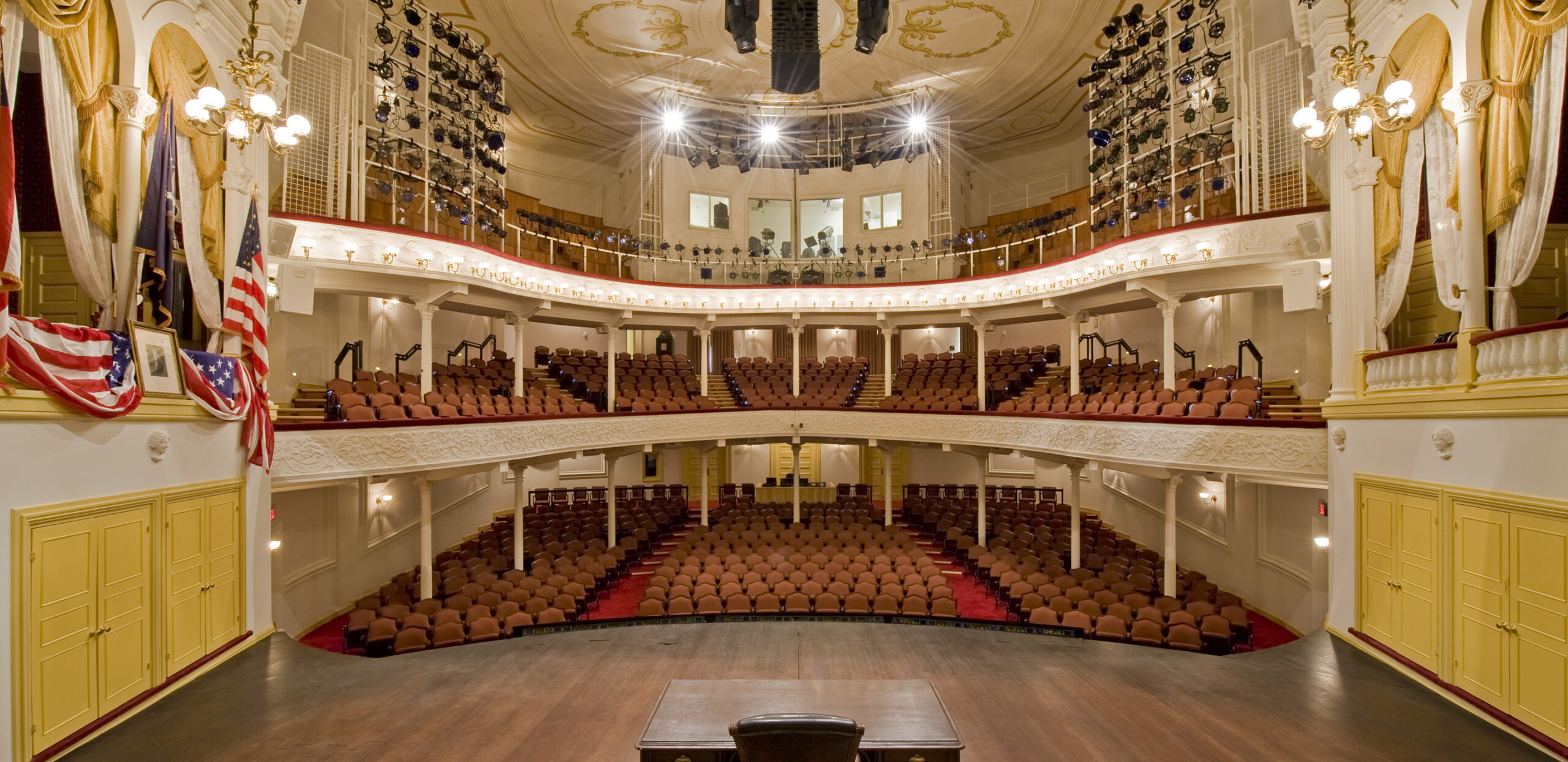This is a detailed photograph taken from the stage of Ford's Theater, the historic venue where President Lincoln was assassinated. The vantage point offers an unobstructed view of the ornate interior, characterized by its cream-colored ceilings adorned with painted designs and supported by white columns. The stage itself is made of vertical brown hardwood slats and features a central wooden desk with a matching chair behind it. Flanking the stage are white walls with yellow doors and booths draped with American flags, including the famous booth where Lincoln was shot, identifiable by the mural of Lincoln and the American flags.

The seating area extends across three levels. The first level consists of rows of brownish, orangish wooden chairs on red carpeted floors, while the second level is elevated slightly above with simpler seating. The third level, positioned highest, houses an array of modern lights aimed downwards at the stage and a projection room area in the center. Across all levels, intricate design elements contribute to a rich historical ambiance, now devoid of any audience, capturing a serene, empty theater space.